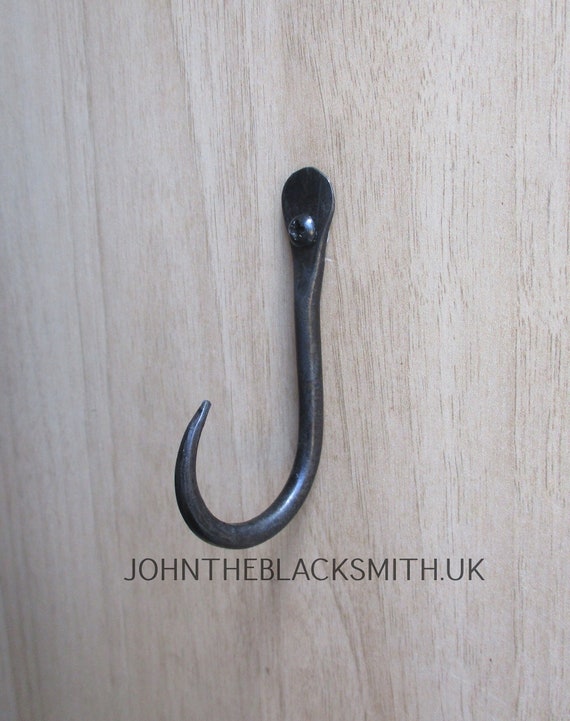The advertisement features an up-close photograph of a simple, curved, black metal wall hook screwed into a light, vertically-grained blonde wooden panel. The hook, centrally positioned in the image, is secured with a phillips head screw and sports a shape reminiscent of a fish hook, with a pressed metal appearance that widens and narrows before curving into the hook. The photograph, minimalist and Shaker-style, comprises only the tan hue of the wood and the grayish-black of the hook. Below the image, in small uppercase black font, it reads "JOHNTHEBLACKSMITH.UK".